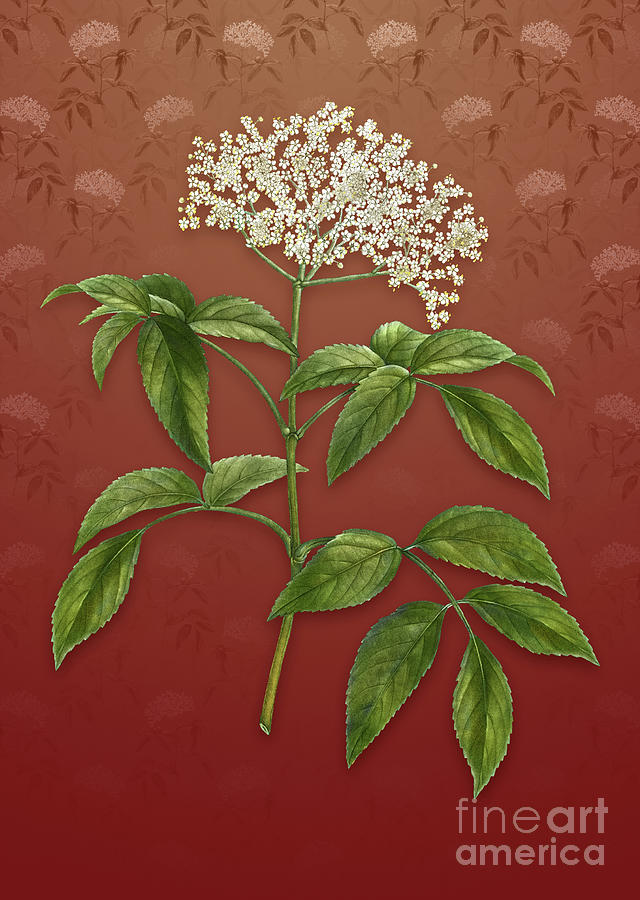This image is a striking piece of graphic art that features a deep maroon to light red ombre background reminiscent of a painting. The background begins as a solid red at the bottom and gradually lightens towards the top. Throughout the upper half of the background, there are faintly visible illustrations of leaves and flowers, creating a subtle layered effect. The central focus is a prominent green stem adorned with clusters of tiny white flowers, resembling a baby's breath plant. The stem showcases four areas where these small flower bunches emerge, surrounded by full, jagged-edged green leaves. The artwork is detailed and intricate, drawing the viewer's eye upward along the central stem. At the bottom right corner, in lighter red text, the words "Fine Art America" are delicately inscribed, anchoring the piece and providing a sense of authenticity and brand. This detailed and layered description captures the richness and complexity of the image, blending the elements provided by different observers into a cohesive and vivid portrayal.